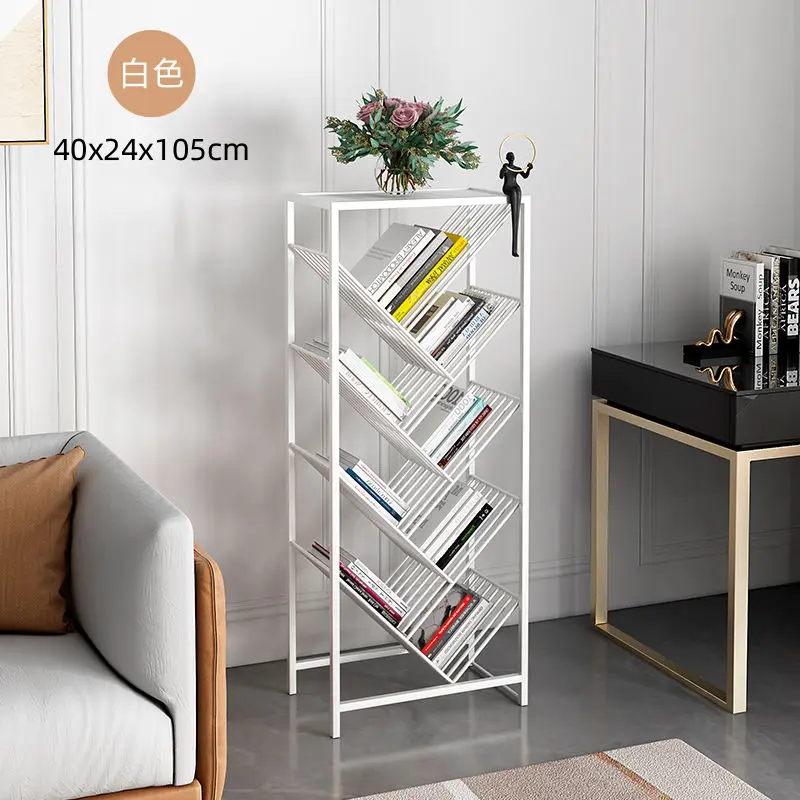This image showcases a part of a home interior with a distinct and modern wire storage rack serving as a bookshelf. The white metal rack, characterized by its staggered shelves arranged in a zigzag pattern, is centrally positioned against a lined off-white wall. The shelves hold various books laid at 45-degree angles, creating a dynamic display. Atop the rack sits a vase, filled with green stems and vibrant red roses, and a small black figurine. To the left of the bookshelf, a brown and gray armchair adorned with a brown pillow is partly visible, while an end table with a chrome-looking brown rim and black top is situated nearby. Additionally, a desk holding more books can be seen on the right side of the image. The floor beneath is gray and a small section of a rug appears at the bottom right corner, completing the cozy room setting.